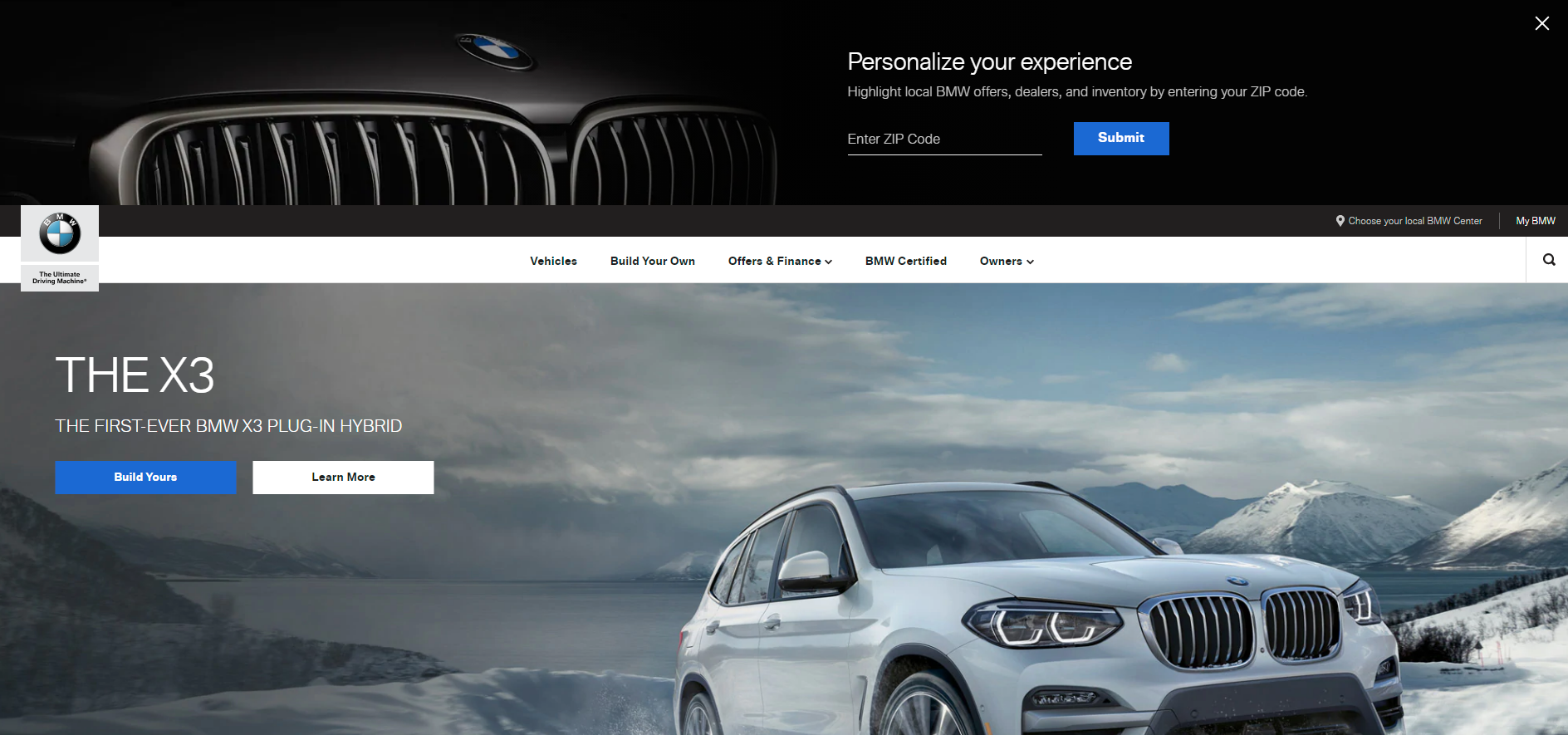The image features a sleek BMW advertisement with a prominent black border at the top. Dominating the upper section is a partial front view of a BMW, showcasing the iconic hood, grille, and the distinguished BMW logo. Above the car, the text reads "Personalize Your Experience: Highlight Local BMW Offers and More by Entering Your Zip Code," accompanied by an input box labeled "Enter Zip Code" and a bold blue button labeled "Submit." Below this header, a navigation menu offers options including "Vehicle," "Build Your Own," "Offers and Finance," "BMW Certified," and "Owners."

Further down, the ad spotlights a BMW SUV angled slightly to the right, displaying the passenger side while obscuring the driver’s side. This vehicle is set against a breathtaking snowy mountain landscape featuring a frozen lake in the background. The atmospheric scene is shrouded in fog and under a canopy of grey clouds. The text below the image introduces the vehicle as "The First-Ever BMW X3 Plug-In Hybrid." The call-to-action includes a blue button labeled "Build Yours" and a white button labeled "Learn More."